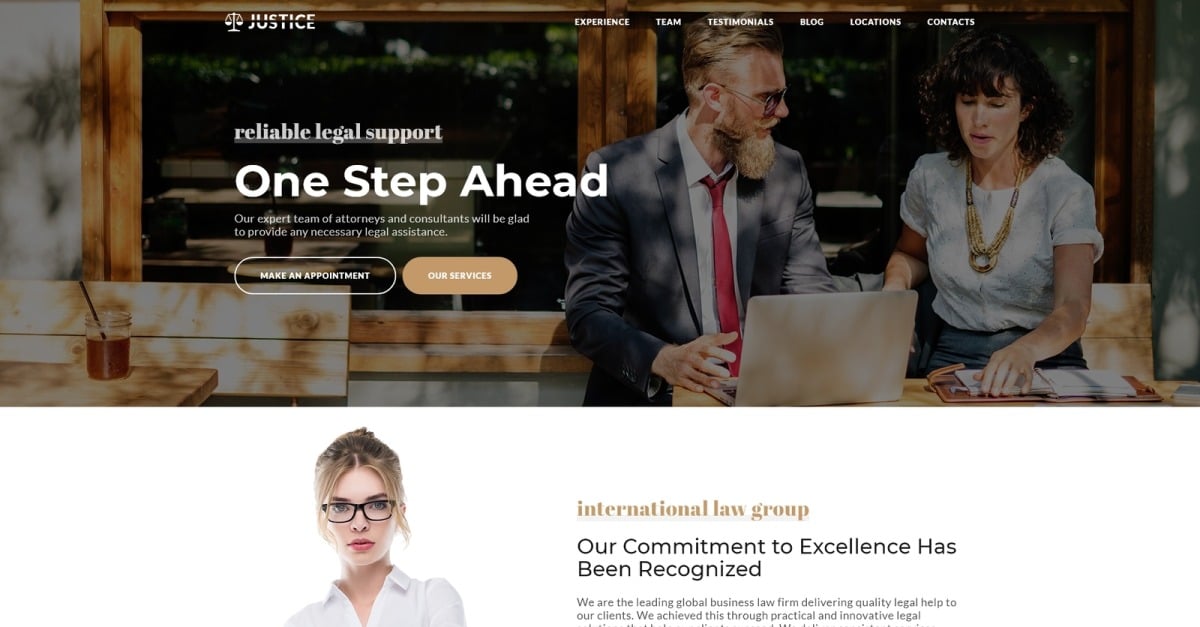The image appears to be a snapshot from a professional website, showcasing the services of a legal firm. The top banner reads “JUSTICE” in bold white letters, accompanied by an image of balanced scales symbolizing fairness and equity. Below this, the tagline “Reliable Legal Support One Step Ahead” is prominently displayed. The website highlights that their expert team of attorneys and consultants is ready to provide any necessary legal assistance.

In the middle section, two interactive buttons are visible: the first is transparent, allowing the background image to show through, with the text “Make an Appointment.” The second button is a beige color, labeled “Our Services.” Above these buttons, there are navigation menus in white text, including options such as Experience, Team, Testimonials, Blog, Locations, and Contracts.

The image features a man seated at a table, engaged in conversation with a woman. The man is wearing sunglasses, a red tie, a white shirt, and a black suit coat. He has a beard, a mustache, and slicked-back hair. Opposite him, the woman has curly black hair, a necklace, and a white shirt. They are both focused on an open laptop in front of them.

Below the image, the text “International Law Group” appears, followed by the phrase, “Our commitment to excellence has been recognized.” Next to this text is a picture of a woman with dark-rimmed glasses and her hair styled up, lending a sense of professionalism and expertise to the scene.